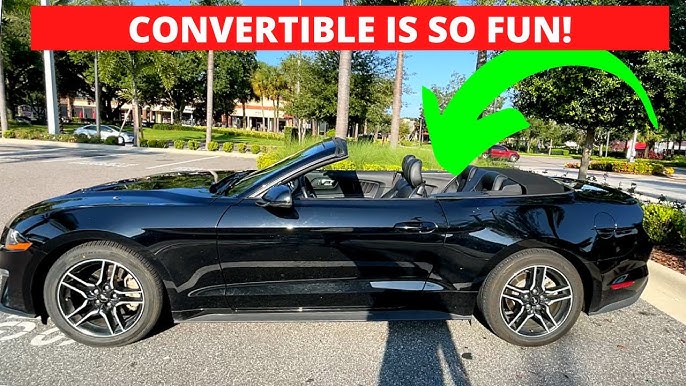In this photograph, a sleek black convertible, possibly a Corvette, takes center stage, facing toward the right with its front end slightly off the bottom left edge of the frame. The convertible, parked in an open parking lot with a gray cement surface speckled in white, appears shiny yet a bit dirty. Spanning the top of the image, a red banner with white text in all caps enthusiastically declares, "CONVERTIBLE IS SO FUN!" A prominent green arrow curves from the top right, pointing toward the back of the convertible.

Surrounding the car, the scene reveals a parking lot bordered by light-colored curbs and green shrubs. In the left distance, there's an asphalt road with another car traveling on it. Across this road lies a green grass field and a long brown brick building, partially obscured by trees and more parked cars. Additional trees and cars can be seen further right, beyond another street that frames the right side of the image. The overall setting exudes a bright, clear day, with a vibrant blue sky and lush greenery, making for a visually engaging and picturesque backdrop.